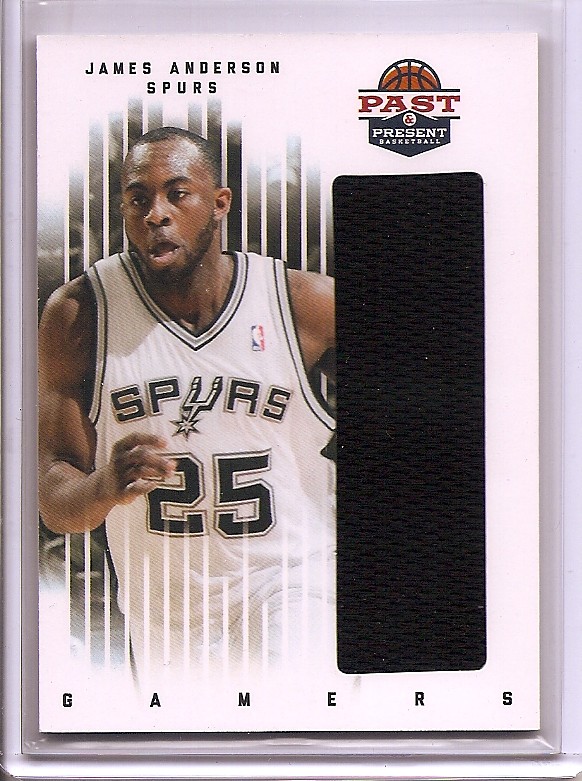The image is a detailed basketball sports card featuring James Anderson of the San Antonio Spurs. The card prominently displays Anderson, a muscular African American player with short-cropped black hair and a chinstrap beard, mid-action, wearing a white Spurs jersey with black lettering and the number 25. Situated on the left side, Anderson's intense expression and sweat suggest he is actively playing. The upper right corner features a logo with a basketball and text in red, blue, and white that reads "Past, Present, Basketball." Below this logo, there is a large black rectangle. The text "James Anderson Spurs" is positioned in the upper left corner. The whole card is framed in white, and "GAMERS" is spelled out with spaced-out letters at the bottom, completing the composition with a cohesive design that emphasizes both the player and the branding.